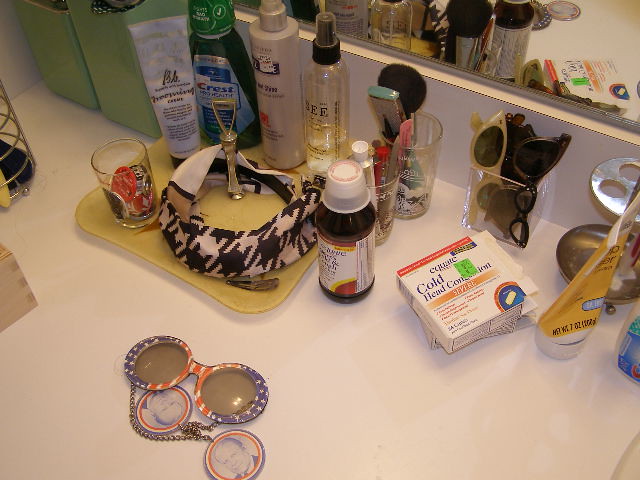This photograph, likely taken in a bathroom, captures a white countertop with a variety of personal items meticulously spread across it. Positioned in the corner of the countertop, the upper left and upper right corners of the image reveal parts of the wall and the lower edge of a mirror, framing the scene.

In the bottom left corner of the photo, a pair of sunglasses adorned with the American flag pattern and fitted with slightly dark, round lenses rests. At the center of the countertop sits a distinctive yellow tray with rounded corners, holding an assortment of items: four bottles of beauty products, a small glass filled with what appears to be badges or bottle caps, and a headband featuring a bold black and white houndstooth pattern.

To the right of the tray are two glasses containing various makeup application tools and possibly nail polish, accompanied by a small bottle of medicine placed in front of them. Adjacent to these, a clear plastic container houses three or four additional pairs of sunglasses. In front of this container, two boxes of cold medicine are neatly stacked atop one another, completing the organized yet bustling tableau of everyday essentials.